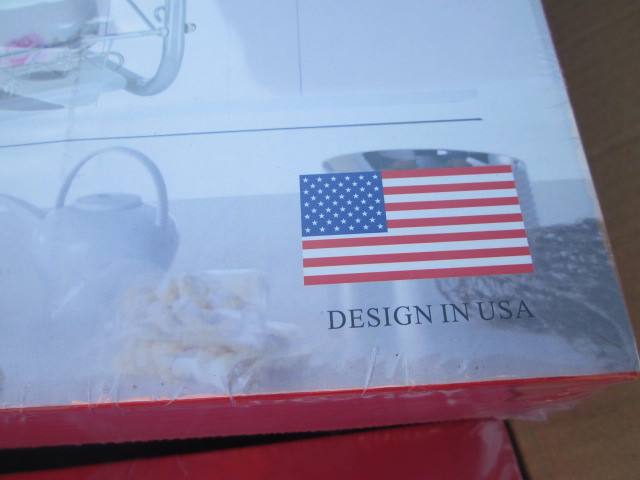The image depicts the lower right corner of a rectangular product box, viewed from a slightly downward angle. The box, wrapped in clear shrink wrap, is positioned so that the corner tilts diagonally from just above the bottom right of the frame to the left. The background is a brownish color in the top right corner of the frame. The box itself has a solid red bottom side and a whitish background. On the top of the box, there is a label featuring an American flag with the text "Designed in USA" beneath it. A white teapot is centrally positioned in the left part of the visible section, with its spout pointing towards the left side of the frame.